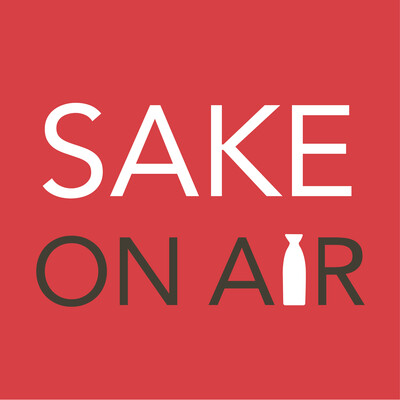The image is a square poster with a striking red background featuring bold text. In large white capital letters, the word "SAKE" is prominently displayed in the center. Directly beneath it, in a smaller and thinner black font, the phrase "ON AIR" is written. What's particularly notable is the letter "I" in "AIR," which is creatively stylized to resemble a tall white sake bottle, complete with a funnel-shaped opening. The entire composition of the words is centrally aligned, suggesting a clean, focused design. The poster creates a simple yet impactful visual, possibly indicating a broadcast or media-related theme, as emphasized by the "ON AIR" text. The colors predominantly used are red for the background, white for the word "SAKE," and black for "ON AIR," with the stylized sake bottle adding a unique touch.